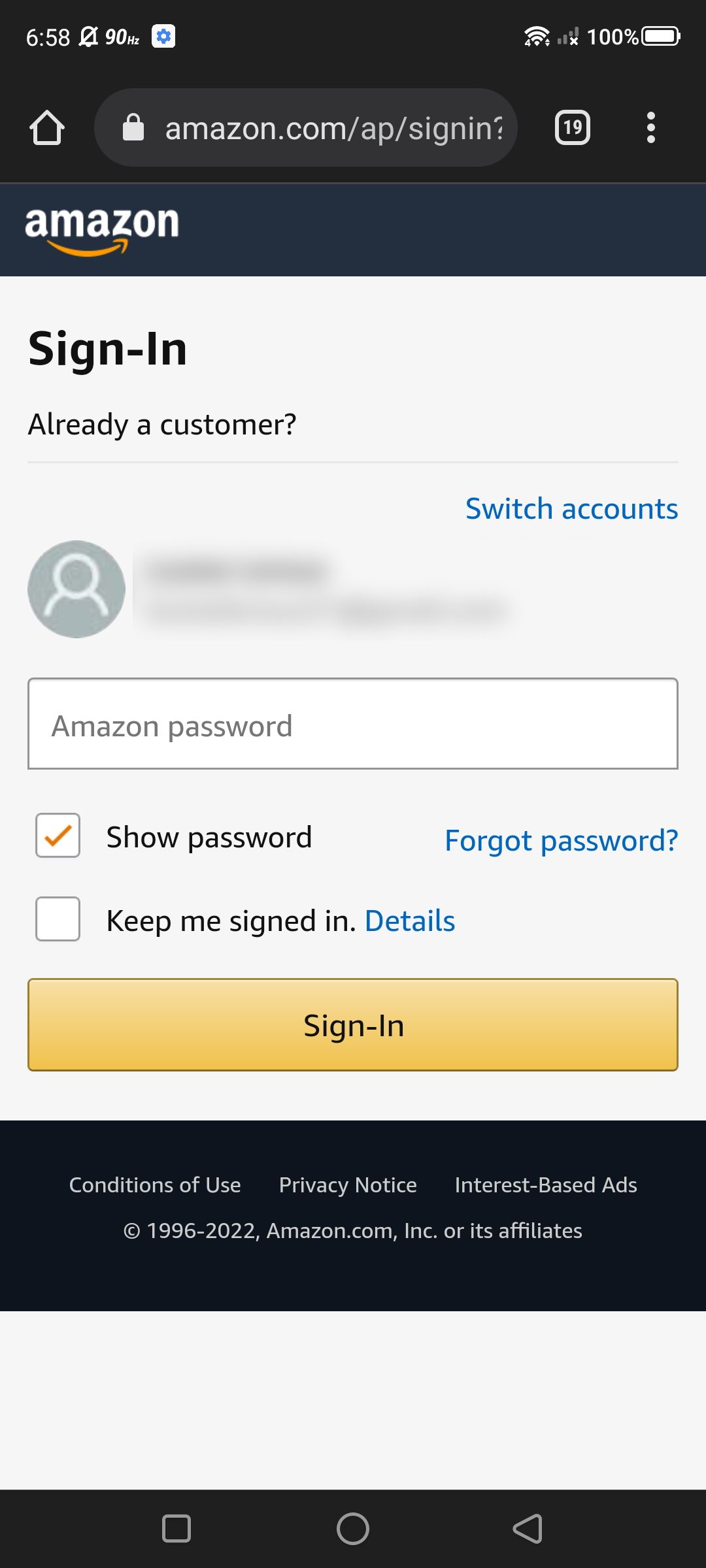The screenshot displays a smartphone screen showing the Amazon sign-in page. The screenshot was captured at 6:58 AM, indicated by the time at the top of the screen. The phone has no service bars but shows a 100% battery level and the alarm is turned off.

At the top, the notification bar includes the signal strength indicator, battery status, and a home button. There are three dots on the right side of the screen for additional options. A circled number '19' appears to the right of the "Amazon.com sign in" text.

The main section of the screen displays the Amazon logo and a light gray circle containing a blurred profile image. Below this, there's a text box for the Amazon password with two options: "Show password" (which is ticked) and "Forgot password?". An unticked box labeled "Keep me signed in" is also present.

At the bottom of the screen, there is a yellow "Sign In" button. Below this button, additional options read as "Already a customer? Switch accounts." There's also text displaying "Conditions of Use," "Privacy Notice," and "Interest-Based Ads," followed by the copyright statement "1996-2022, Amazon.com, Inc. or its affiliates."

Finally, the navigation bar at the very bottom of the screen includes the standard square, circle, and triangle buttons for navigation.